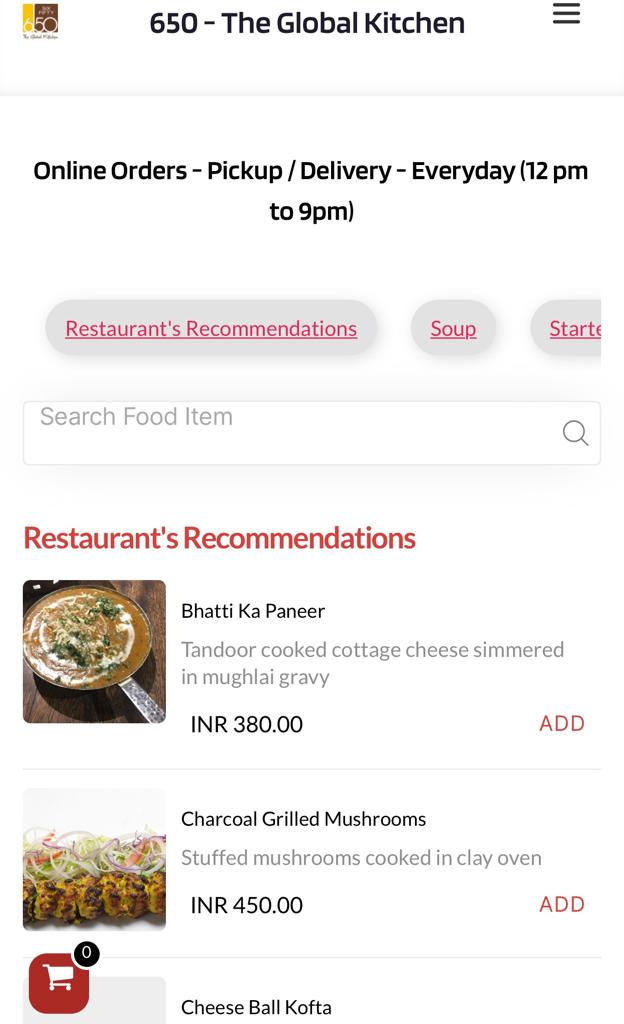**Screenshot of the Global Kitchen Application Menu**

This screenshot showcases the interface of the Global Kitchen application. At the top of the screen, the header reads "650-The Global Kitchen," accompanied by the Global Kitchen logo positioned to the left and a Hamburger Menu icon to the right. Directly below the header, the application displays the message "Online Order/Pickup and Delivery Every Day from 12 p.m. to 9 p.m."

The menu is divided into various sections, highlighted with capsules that feature red text. The sections include "Restaurant Recommendations" and "Soup and Starters" with the "Starters" label partially cut off on the right side of the screen, indicating a slideable menu.

A search field labeled "Search Food Item" is positioned below the main categories. Under "Restaurant Recommendations," two dishes are prominently displayed:

1. **Bhatti Paneer:** An image of the dish, presented as a delicious curry in a silver pan, garnished with spices and cream. The description reads, "Tandoor cooked cottage cheese simmered in Mughlai gravy," priced at INR 380.00 (with INR referring to Indian Rupee). To the right of this description is a red "Add" button.

2. **Charcoal Grilled Mushrooms:** A sumptuous dish of stuffed mushrooms cooked in a clay oven, priced at INR 450.00. This item also includes an "Add" button to the right.

At the bottom of the display, the shopping cart is visible, currently showing a zero inside a black circle, indicating no items have been added yet. Below the displayed recommendations, another menu item titled "Cheese Ball Kafta" is visible but has not been selected.